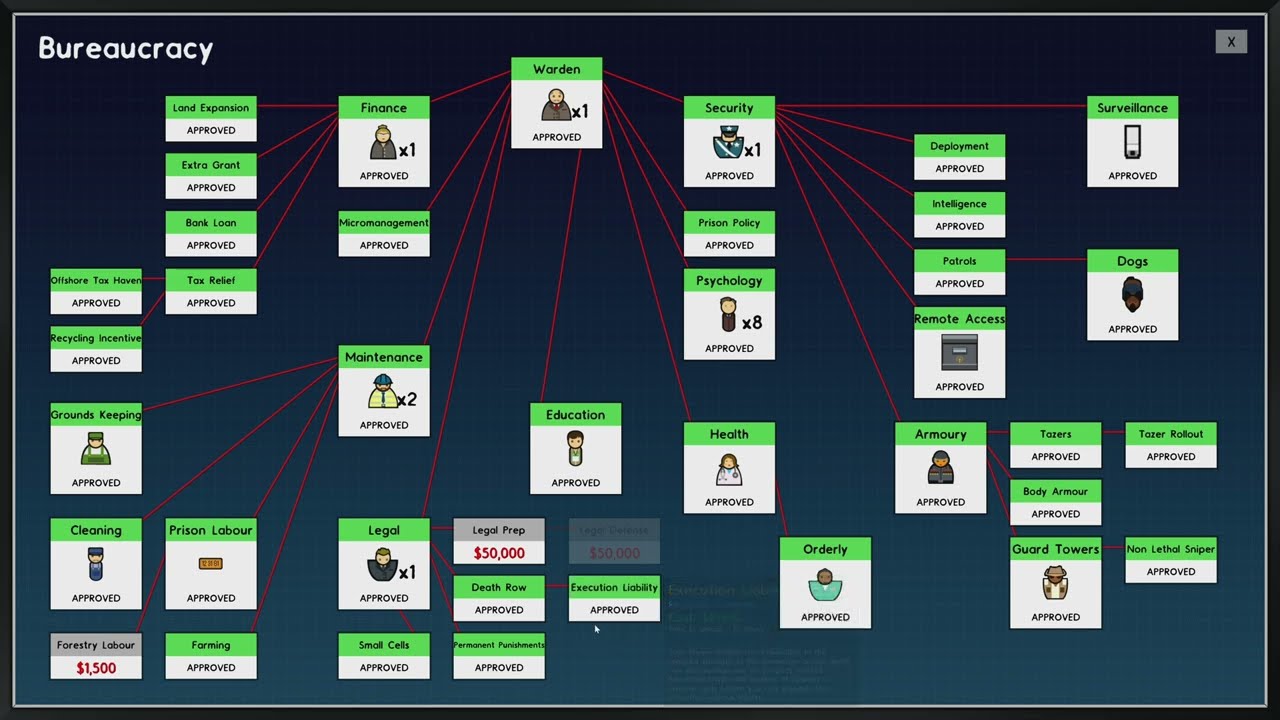This image depicts a complex diagram titled "Bureaucracy" in the top left corner of a dark blue background. It resembles an educational slide or a screencap from a video game. At the center, there is a prominent box labeled "Warden," which acts as a hub connecting to various other boxes and categories, indicative of different roles and responsibilities.

Each box contains specific titles and sometimes icons with approval stamps, such as "Security" featuring a police officer emoji with "x1 Approved." Key categories connected to the Warden include Finance, Land Expansion, Bank Loan, Tax Relief, Health, Orderly, Education, Legal, Maintenance, and Prison Labor. Subcategories under these major areas detail further responsibilities and approvals, like "Groundskeeping," "Cleaning," "Recycling Incentive," "Forestry Labor," and "Prison Policy."

Additional titles such as "Farming Approved," "Remote Access," "Armory," "Dogs," "Surveillance," and "Department Intelligence" are also displayed, demonstrating the extensive reach of the bureaucratic structure. The diagram visually organizes each role and task into interconnected blocks, suggesting a detailed mapping of hierarchical or functional duties. A noticeable gray "X" in the corner indicates the option to close the interface.

Overall, the detailed construction of this diagram provides an encompassing view of the key functions and interrelations within a bureaucratic or managerial setting, likely in the context of a game or an instructional aid.